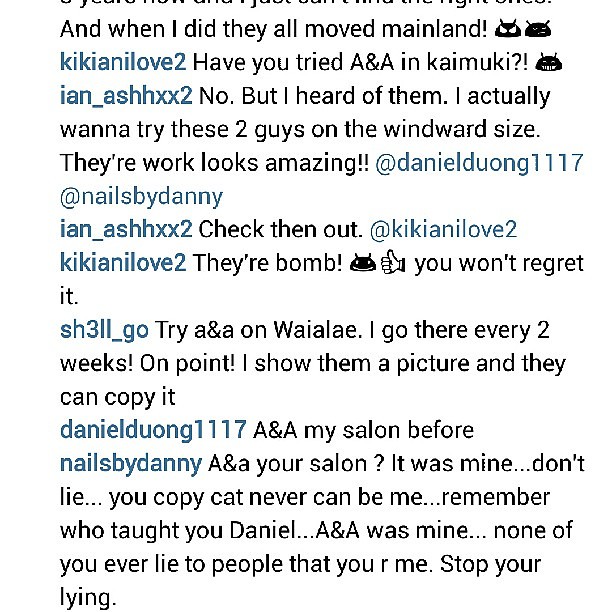The image is a screenshot of a text conversation on a social media messaging app, likely Instagram or Facebook. The conversation is between Kiki Yani Love 2 and Ian Ash XX2, who are both in Hawaii, specifically on the island of Oahu. The text appears in black on a white background without any distinct objects. 

The discussion revolves around nail salons and artists on the island. Kiki initiates the conversation by asking Ian if he has tried A&A or Kaimuki. Ian responds that he has heard of them but hasn't tried them yet. Instead, he shows interest in two artists on the Windward side, Daniel Duong and Nails by Danny, whose work he praises highly. Kiki agrees that they are excellent and assures Ian that he won't regret trying them out.

The conversation also includes a mention of going to A&A salon in Wailea every two weeks, where the service is highly rated for replicating designs shown by customers. There is a contentious exchange where it appears that Nails by Danny claims ownership over A&A, accusing Daniel of copying and lying about being the originator.

Overall, the screenshot captures a detailed exchange with recommendations and personal opinions on local nail salons and their services, highlighting both collaboration and rivalry in the beauty community.